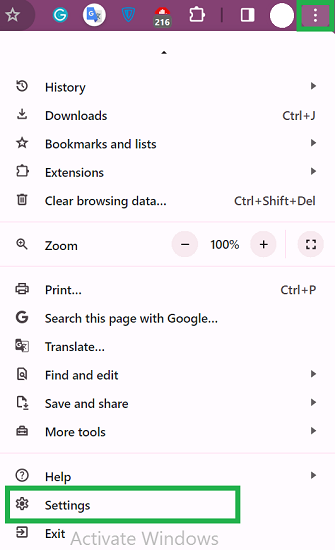A detailed screenshot shows a user's smartphone displaying a menu with a purple ribbon running across the top of the screen. The ribbon contains various icons, likely representing different app functionalities. Below the ribbon, the content is presented on a clean white background featuring a vertical list of options in black text.

The listed options include:
1. **History**
2. **Downloads**
3. **Bookmarks and Lists**
4. **Extensions**
5. **Clear Browsing Data**
6. **Zoom**
7. **Print**
8. **Search This Page with Google**
9. **Translate**
10. **Find and Edit**
11. **Save and Share**
12. **More Tools**
13. **Help**
14. **Settings**
15. **Exit**

Adjacent to each term is a corresponding icon: a download icon for "Downloads," a star for "Bookmarks and Lists," a trash can for "Clear Browsing Data," a magnifying glass for "Zoom," and a printer for "Print," among others.

The "Settings" option and its associated settings icon are selected and highlighted in green, indicating the current focus. Below the "Exit" option, near the bottom right of the screen, is a subtle message in pale gray text that reads "Activate Windows."